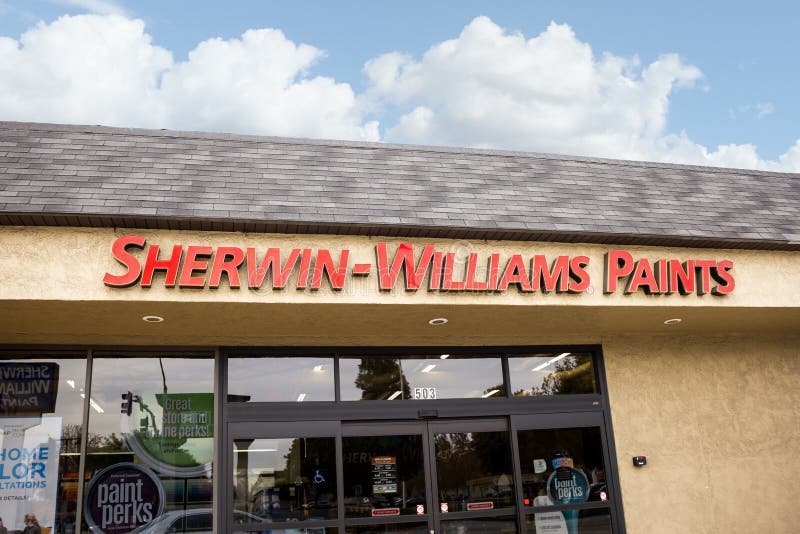The image showcases a Sherwin-Williams paint store set against a backdrop of a vibrant blue sky with scattered fluffy white clouds. The building features a brown roof and prominently displays "Sherwin-Williams Paints" in bold red capital letters. Beneath the sign, three lights illuminate the exterior. Visible on the store’s facade is a circular sign with a purple background and the words "Paint Perks" written in white.

The glass entrance doors display several signs and posters. A large poster on the left door reads "Home Floor Installations" in blue lettering. Another sign announces "Great In-Store Perks" on a green circular background with white text. Above the entrance, the address "503" is clearly marked in black letters at the top of a window.

One of the doors is adorned with a blue and white handicapped sign, and next to it, a posting of the store's hours of operation. A red and white sticker indicates that the doors are automatic. On the right-hand side, another circular sign with a blue background reads "Paint Perks" in white letters, reinforcing the store’s loyalty program.